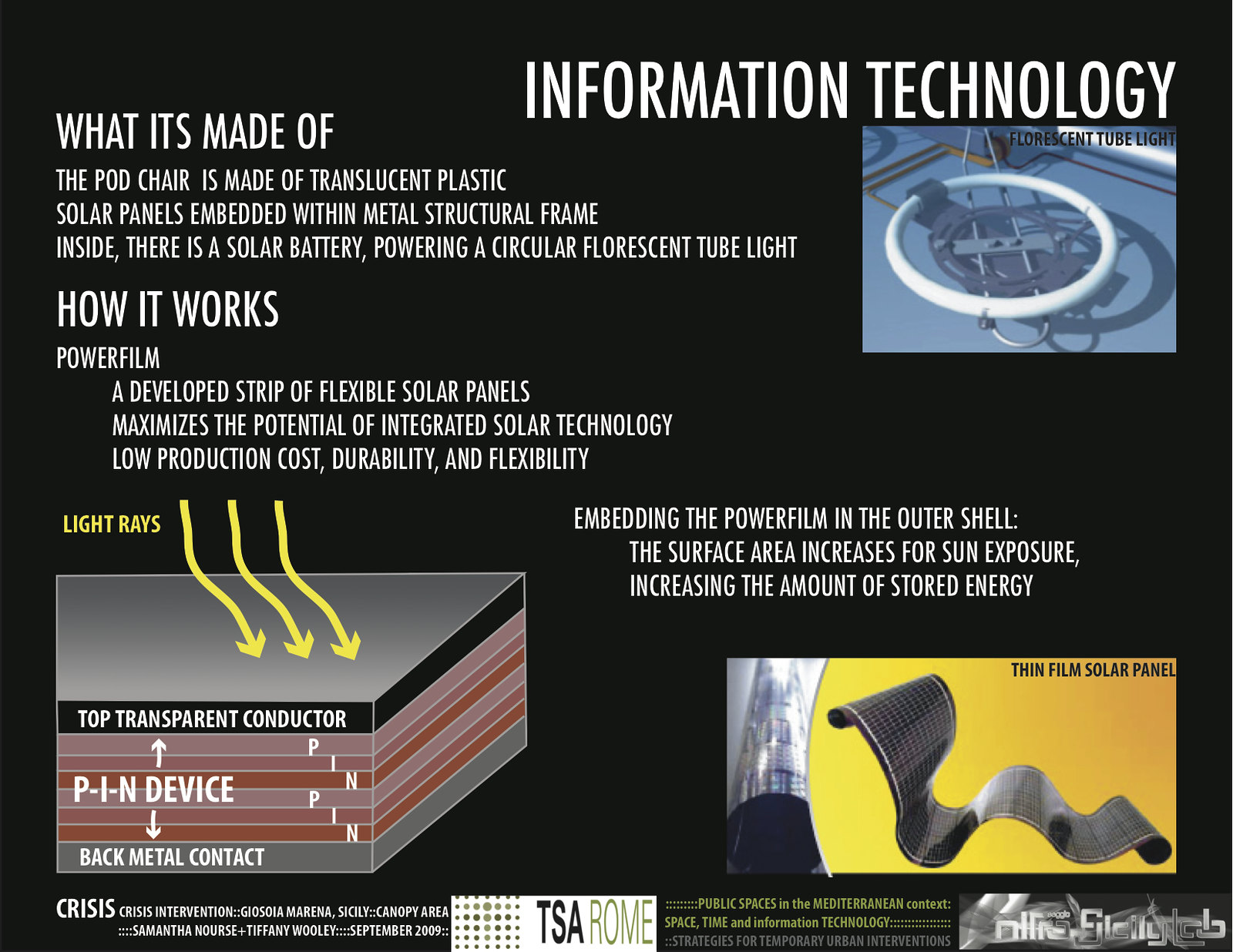The image is a black-background flyer or slide, heavily centered around Information Technology, indicated by large white letters at the upper right corner. Directly beneath this title, the flyer features an image of a circular fluorescent tube light labeled "fluorescent tube light," set against a blue backdrop. To the left, a prominent header reads "What It's Made Of," describing a pod chair constructed from translucent plastic embedded with metal-frame-structured solar panels. The text explains that inside the chair, a solar battery powers the circular fluorescent tube light.

Further down, another header titled "How It Works" details the functionality of integrated solar technology. A diagram accompanies this section, illustrating light rays hitting the surface, which has layers labeled in various colors: a black and grey top transparent conductor, pink and reddish middle layers described as a PIN device, and a grey bottom layer as the metal contact.

At the bottom right of the flyer, another image shows a wavy ribbon-like thin film solar panel, captioned "thin film solar panel." The bottom border of the flyer is dense with additional information, including various logos and text in fine print. There are mentions of "Crisis Intervention," TSA Rome, NILFRA Sicily Lab, and public spaces in the Mediterranean context among others. This section also includes a detailed list of names and dates, such as Geosia Marina, Sicily Canopy Area, and Samantha Knots plus Tiffany Wooley, September 2009.